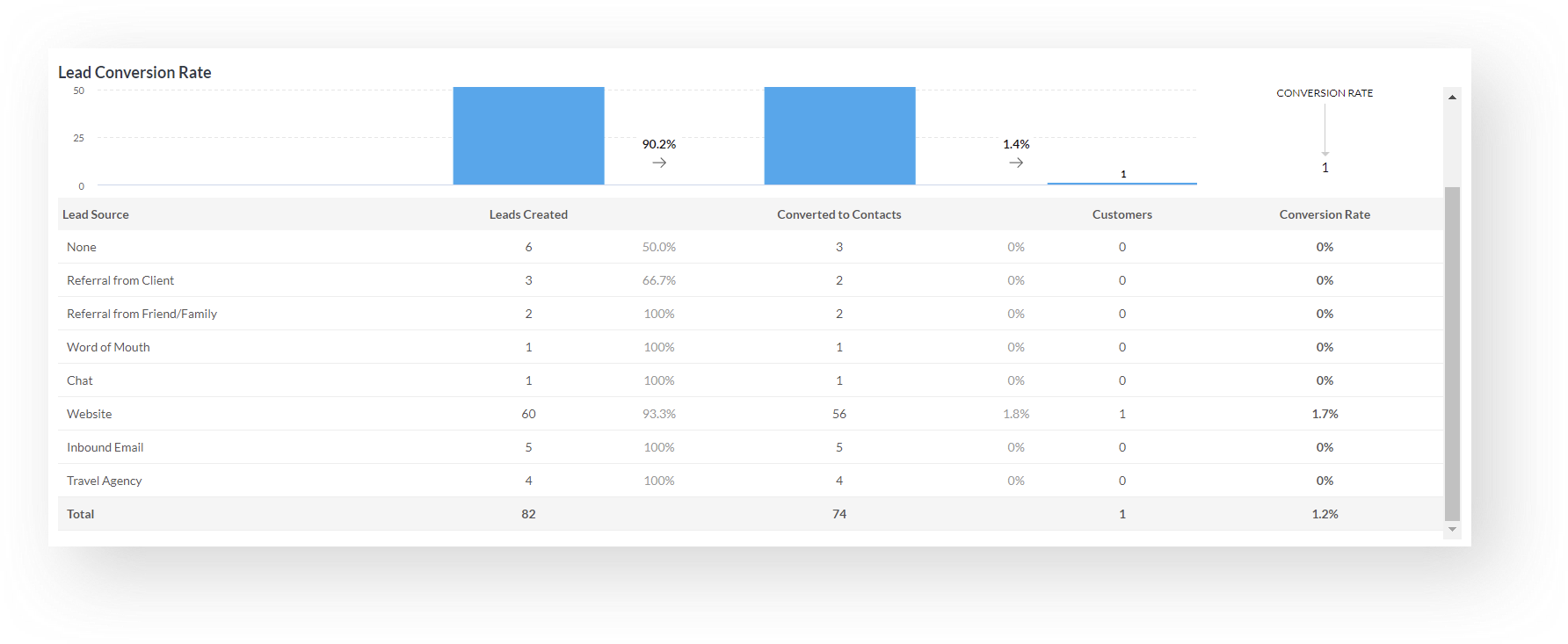The image is a screenshot of a statistics chart from a website. At the top left corner, the title "Lean Conversion Rate" is displayed. Below the title, there are two horizontal bars with a value of "90.2%" positioned between them. An arrow pointing to the right follows this value, indicating a subsequent percentage of "1.4%". Towards the bottom of the image, there is a section titled "Lead Source" with various blurry words listed. The discernible sources include "Name", "Website", "Word-of-mouth", "Chat", and "Travel Agency", each accompanied by their respective percentages, although only some of the percentages are legible.